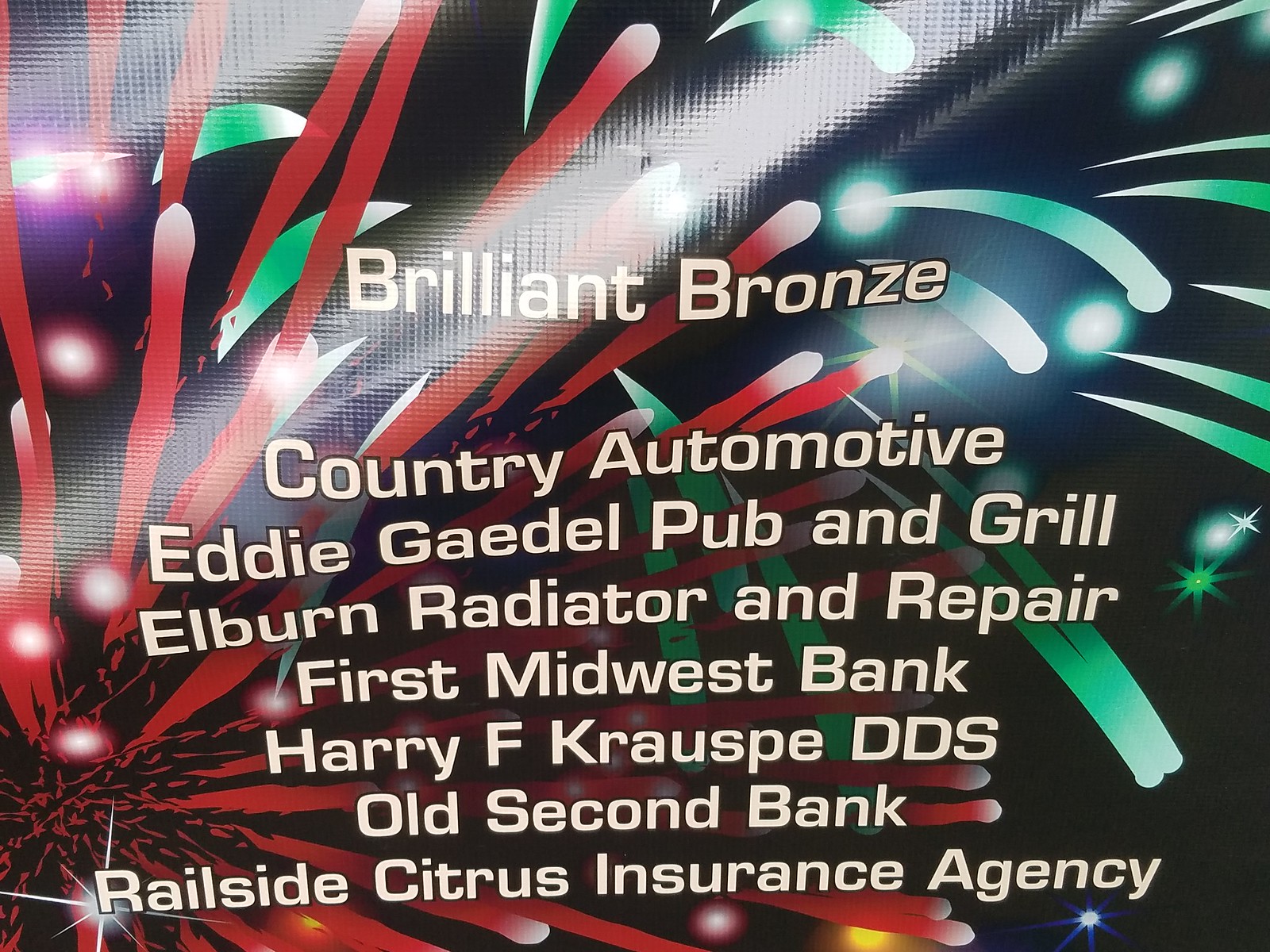This image features a vibrant background resembling a display of red and green fireworks. Overlaid on this dynamic backdrop is a series of businesses and names written in white, sentence-case text, arranged one beneath the other from top to bottom. The list includes "Brilliant Bronze," "Country Automotive," "Eddy Gatel Pub and Grill," "L Burn," "Radiator and Repair," "First Midwest Bank," "Harry F. Krausp, DDS," "Old Second Bank," and "Railside Citrus Insurance Agency." Additionally, there is a noticeable glare in the left diagonal quadrant of the image, which slightly obscures part of the background.